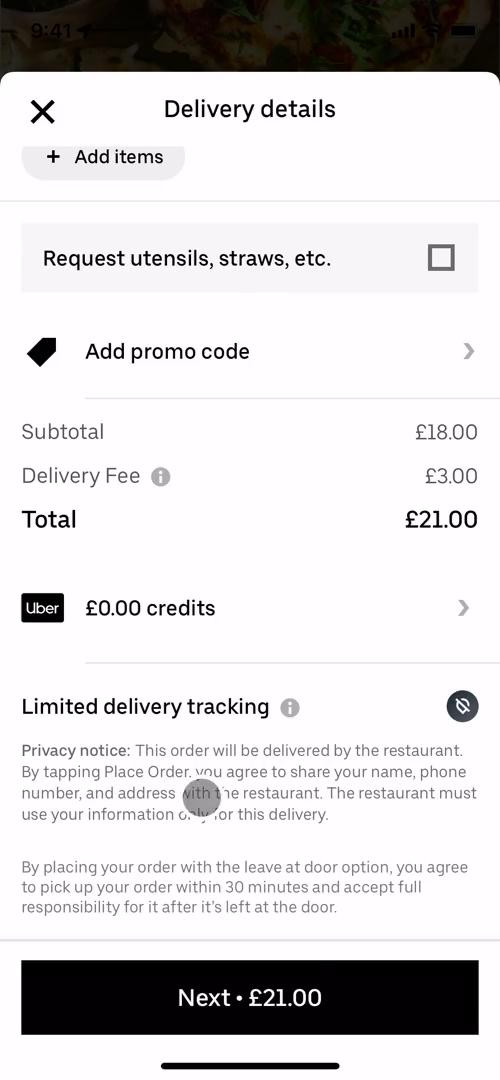Detailed Caption: 

This image showcases a mobile app interface from Uber Eats, capturing an in-progress food order. The background of the top section features a delectable pizza image. The app screen is predominantly white with black text detailing various ordering options and information.

At the very top-left corner, a black 'X' is visible for closing the screen. Below this, the section titled "Delivery details" precedes an option to "Add items." Further down, there is an option labeled "Request utensils, straws, etc.," accompanied by a checkbox to facilitate this request.

Proceeding further, the user is given the option to "Add promo code," with a clickable ticker on the right to expand and enter any applicable codes. The financial breakdown begins with a "Subtotal" listed as £18.00, followed by a "Delivery fee" of £3.00. An information icon next to the delivery fee offers additional details when tapped.

Highlighted in bold text is the "Total," amounting to £21.00, displayed prominently to the right. A subsequent expandable section labeled "Uber" indicates the user has zero Uber Eats credits. Below this, notables like "Limited delivery tracking" and a "Privacy notice" are mentioned.

At the bottom of the screen, a prominent "Next" button is featured, enabling the user to proceed with their order, reaffirming the total cost of £21.00.